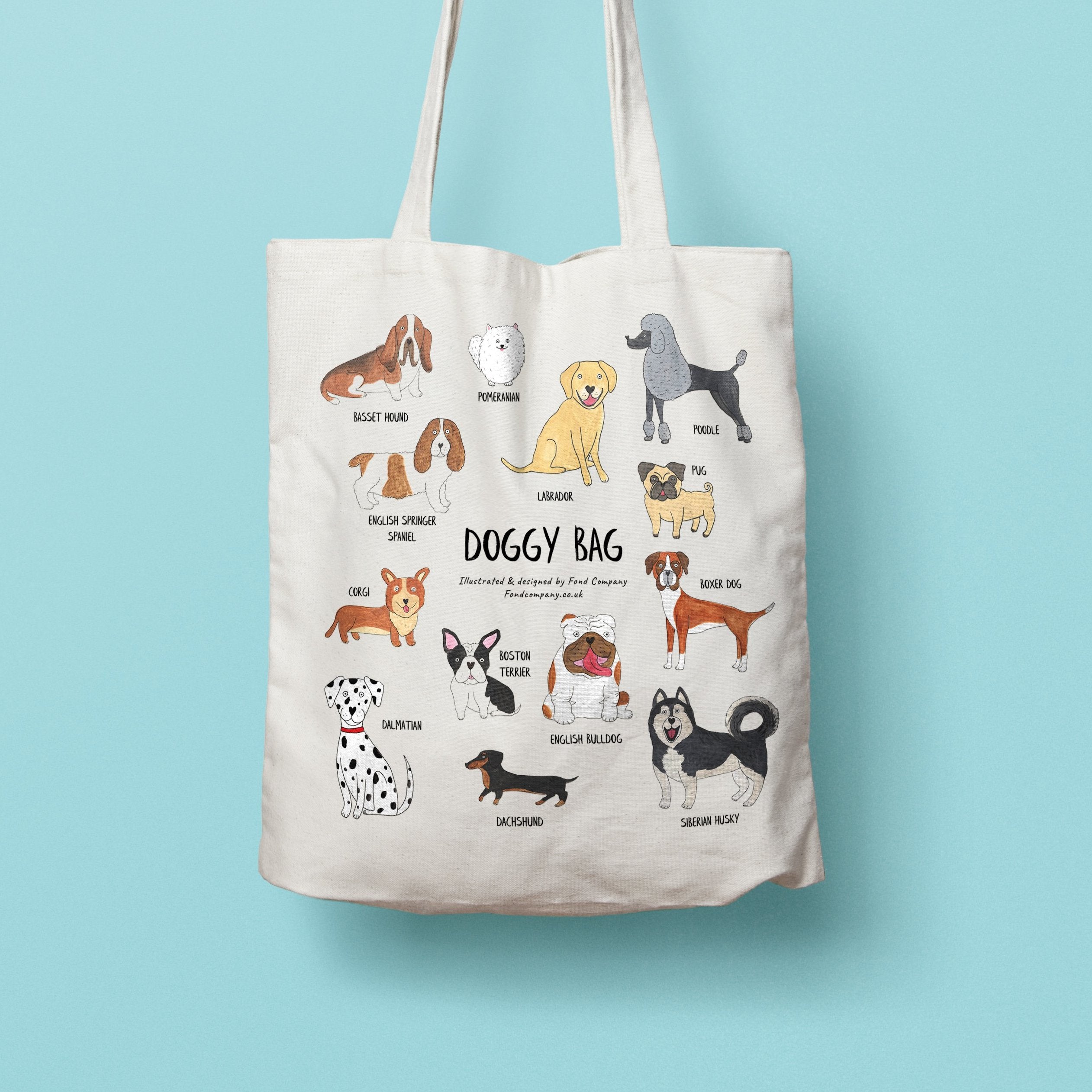The photograph showcases a perfectly square image with a light blue background reminiscent of Tiffany's blue. Centrally positioned is a cream or off-white rectangular canvas tote bag, which appears to be hanging, likely from a peg, as the long, loopy handles are partially visible but cut off at the top. Adorning the bag are numerous charming illustrations of various dog breeds, each labeled accordingly. In bold black text at the center, it reads, "Doggy Bag,” followed by "illustrated and designed by Fawn Company, fawncompany.co.uk."

The detailed illustrations include a range of dog breeds such as a Basset Hound, Pomeranian, Labrador, Poodle, Pug, Boxer Dog, English Bulldog, Boston Terrier, Corgi, Dalmatian, Dachshund, English Springer Spaniel, and a Siberian Husky. Each dog is depicted in a cute, simplistic style with colors ranging from browns and whites to grays. The dogs are either sitting or standing on all fours, all looking forward or to the left, creating a delightful and cohesive design. This canvas tote bag, ideal for shopping trips, combines functionality with an adorable dog-themed aesthetic, making it a perfect accessory for dog lovers.